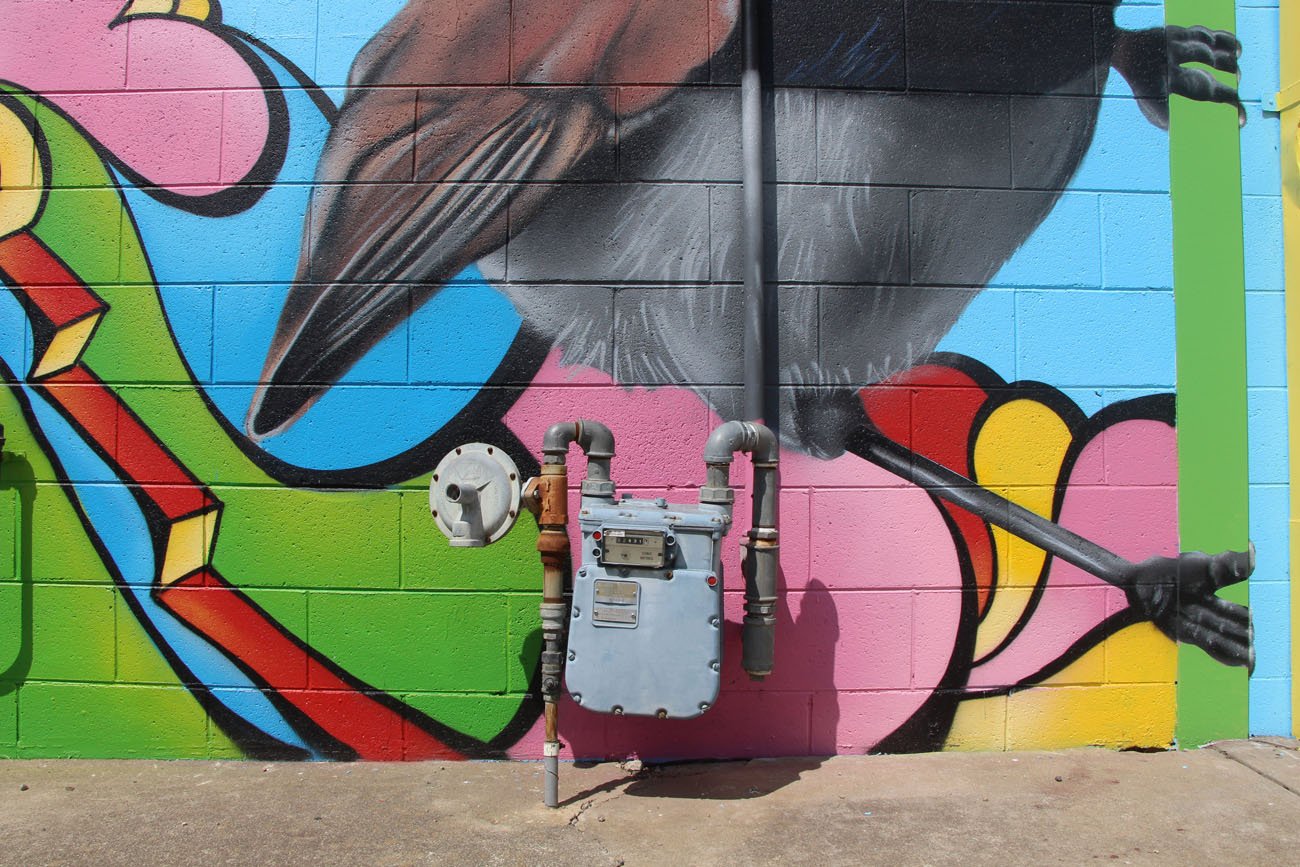This vertical rectangular image captures the side of a building with a vividly painted concrete block wall featuring a striking, large gray bird gripping a green pole. The bird's wings are brown, its belly is white, and its claws are black. Surrounding the bird are splashes of bright colors, including greens, reds, yellows, blues, and pinks, forming an abstract backdrop. Below, the brownish-gray sidewalk borders a gray, metallic mechanism, identified as an energy or water meter. This device, drilled into the ground, features a label on the front and a network of pipes that rise from the base, extend horizontally at the top, then descend back into the wall.